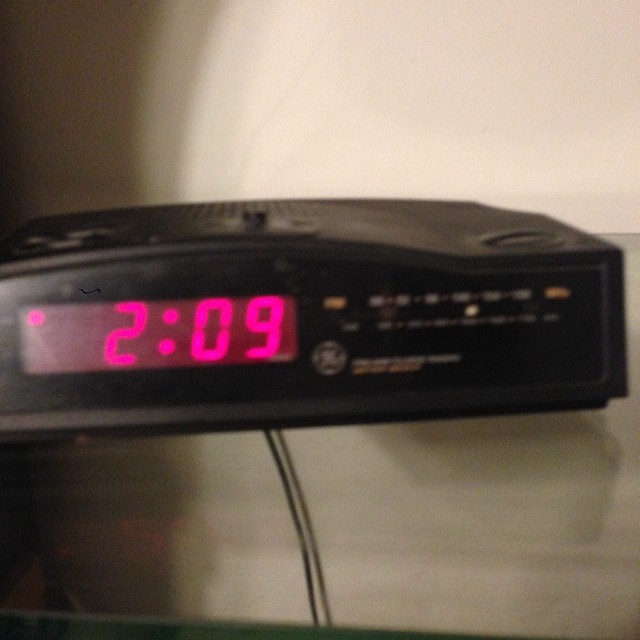This indoor color photograph captures a black, old-style, digital GE alarm clock, likely from the early 90s, placed centrally on a glossy white surface, possibly a glass-topped bedside table. The clock displays the time 2:09 in red glowing numbers with an illuminated 'AM' dot in the upper left. The clock's black frame and body contrast sharply against the white background. The upper left section and lower right portions of the image have shadows. Despite the image's grainy and slightly out-of-focus quality, the thin black power cord descending from the bottom of the clock and trailing towards the bottom of the photograph is recognizable. The clock features an old-fashioned AM/FM radio dial on the right with knobs for volume and station adjustments, as well as buttons on the top surface. Although details like specific radio frequencies and additional text next to the GE logo on the front face are indiscernible due to the blurry capture, the photograph clearly conveys the nostalgic essence of the clock radio, enhanced by the faint semi-reflection on the glossy surface below.